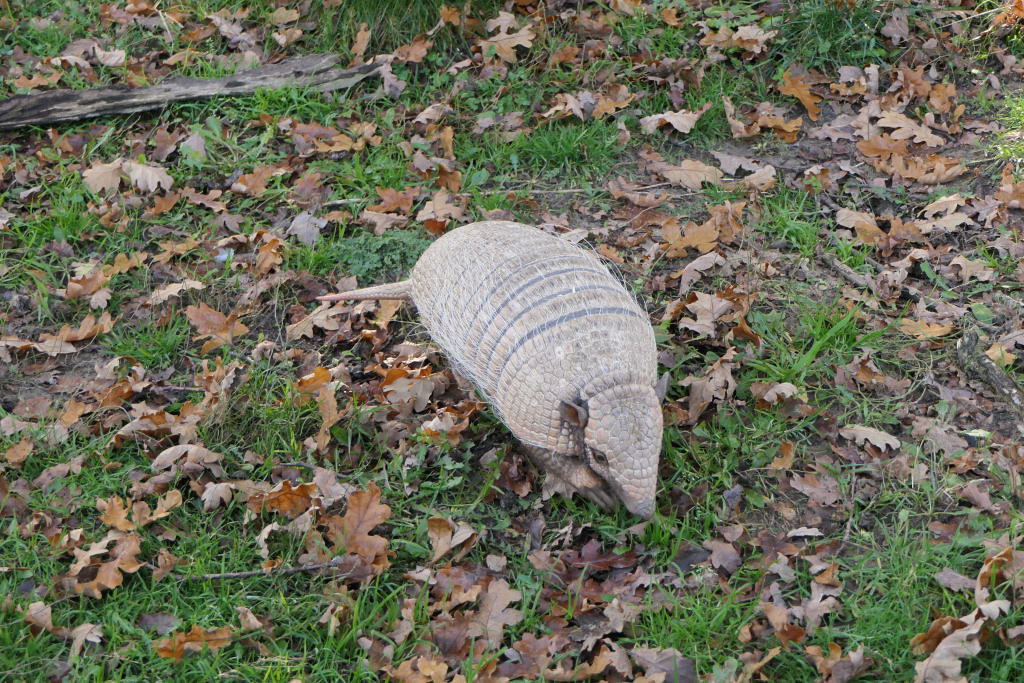In this detailed image, a small armadillo is quietly sitting in a grassy area covered with autumn leaves. The armadillo's body features a light gray, scaly back and front, adorned with distinct darker gray lines. Its small ears and pointy tail also exhibit the characteristic scales. The calm demeanor of the armadillo suggests it is neither aggressive nor frightened, simply relaxing on the ground. Surrounding the armadillo, one can see a fallen twig and various other small branches scattered among the brown leaves and patches of dirt, further enhancing the rustic, natural setting. The scene provides a serene glimpse into the armadillo's tranquil environment, capturing the peaceful essence of this well-groomed animal.